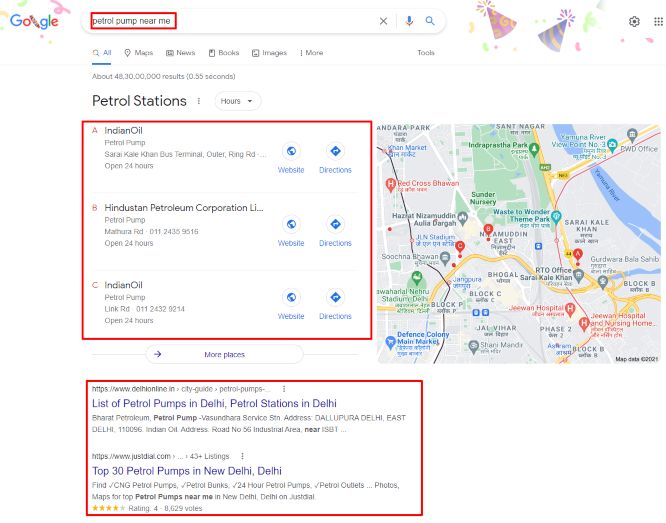A Google search screenshot features a festive, customized Google logo celebrating what appears to be a birthday or similar holiday. In the upper left-hand corner, the celebratory Google logo replaces the standard version. To the right of the logo, the search bar displays the query "petrol pump near me," returning over 48 million results.

Below the search bar, the first section is titled "Petrol Stations," listing three local stations: Indian Oil, Hindustan Petroleum Corporation, and another Indian Oil station. An option to discover more places is also provided.

Further down the results page, there are additional links, including "List of petrol pumps in Delhi" and "30 petrol pumps in New Delhi."

The user has highlighted certain elements of the screenshot with drawn boxes: the search term "petrol pump near me" in the search bar, the "Petrol Stations" section, and the additional links at the bottom, all marked with red squares. The background is predominantly white, providing a clean and easily readable interface.